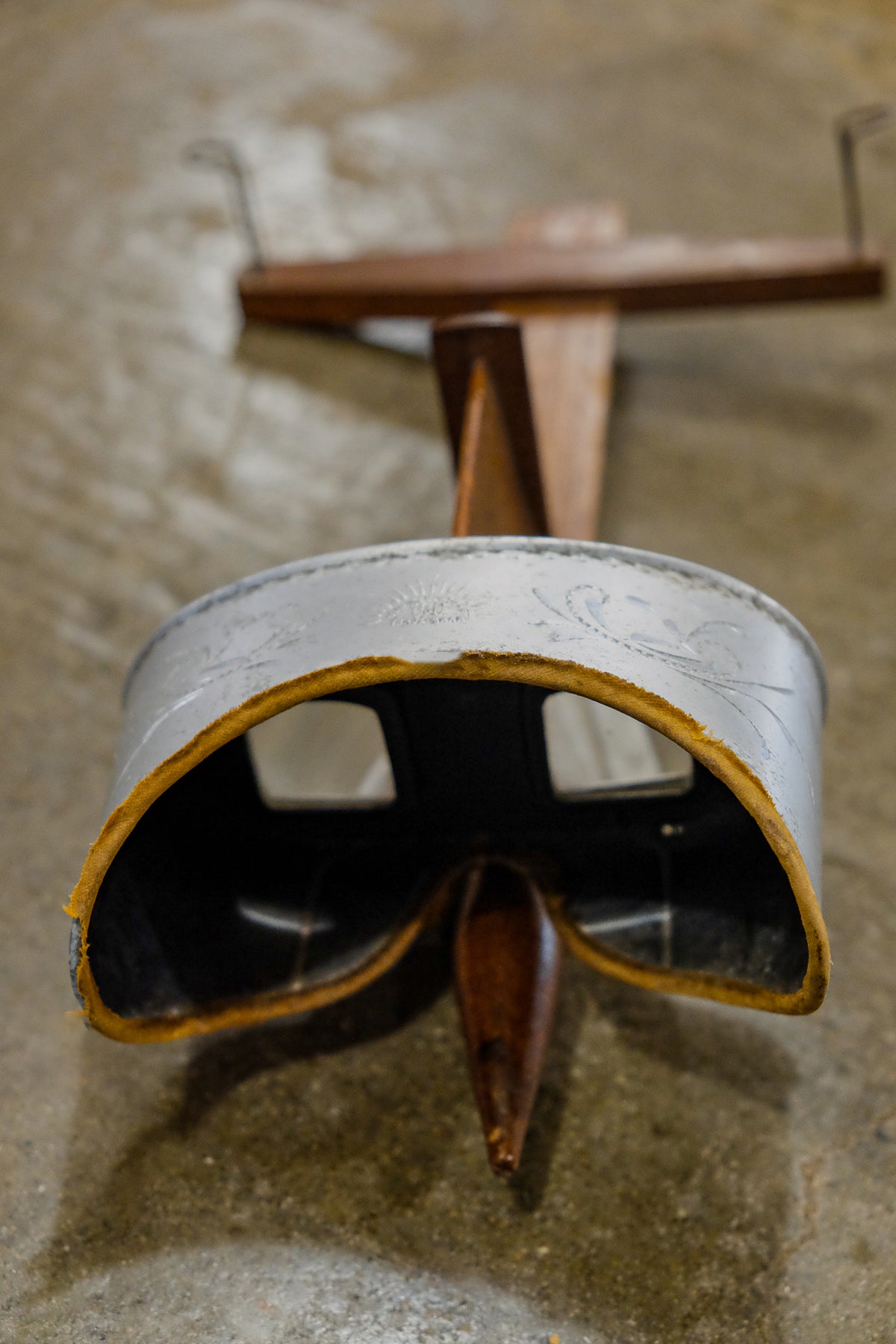The photograph is a vertically oriented, rectangular image, likely taken from a mobile phone. The object depicted rests on what appears to be a dark brown, brownish-gray, or greenish-gray concrete surface. This object is a vintage stereoscope, a device used for viewing two photographs to create a single three-dimensional image.

The stereoscope features a metal faceplate with indentations for cheeks and nose, and curves inward at the top to accommodate the forehead. This faceplate appears to have intricate filigree engravings and is edged with deteriorating yellow fabric, providing a lightly padded rim where a user's face would rest. The eyeholes or viewports are small and square-shaped, allowing the user to peer through to the image.

Extending from the faceplate is a wooden structure, with a central plank forming a T-shape. The distal end of this wooden plank holds a card or photograph, which can be adjusted closer or further from the viewer's eyes. The entire setup suggests a mechanism designed to align each eye with different portions of a stereoscopic image to create a 3D visual effect.

The background of the image is slightly blurred, focusing attention on the antiquated device, which combines both wooden and engraved leather elements, suggesting its historical usage as an entertainment or viewing gadget.